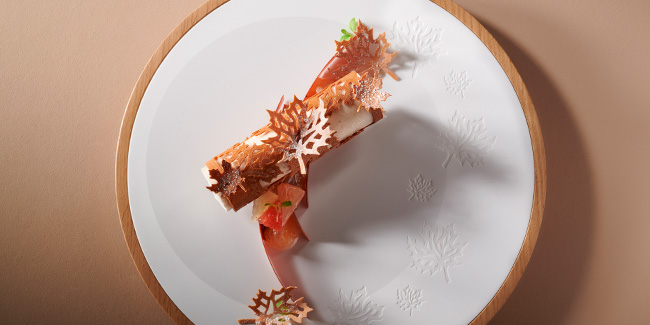The image is a professionally taken, full-color photograph that is horizontally rectangular without a border. The background is a brownish-tan hue, likely indicating a table surface. At the center of the image is a white circular plate adorned with an etched leaf motif, especially noticeable on the right side where a shadow from the plate falls. The plate is encircled by a brown wooden trim that enhances its elegant appearance.

Sitting in the middle of the plate is an exquisite dessert that appears very fancy and intricate. The dessert is brown in color and curved in shape, with a rich white cream filling visible inside. The top of the dessert is decorated with finely cut, leaf-like elements that resemble little leaves or snowflakes, giving it a whimsical and artful presentation. One of these leafy elements is separate and rests at the bottom of the dessert, further adding to its elaborate design. White powder lightly dusts the dessert, enhancing its sophisticated aesthetic.